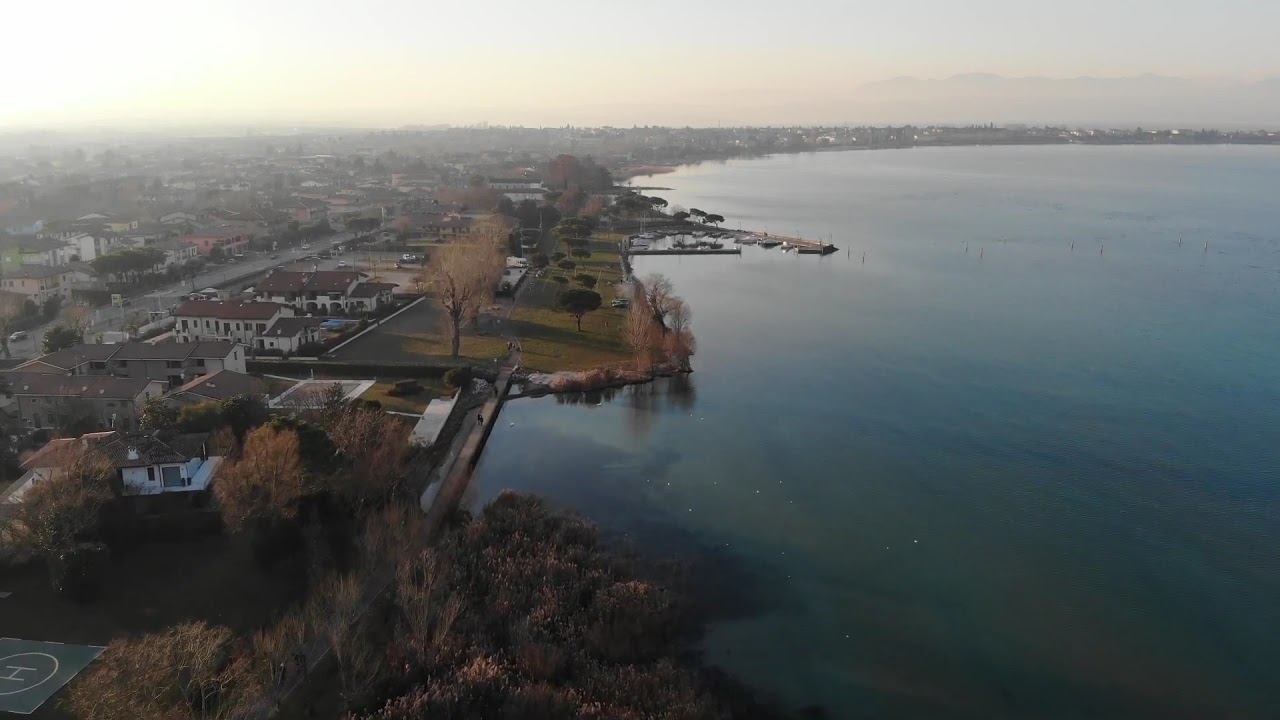This aerial photograph captures a picturesque town on the perimeter of a large, serene body of water, possibly a lake or bay. The town, devoid of skyscrapers, features numerous two or three-story buildings and expansive warehouses near the water. A notable park, rectangular in shape and adorned with trees amidst a grassy area, stretches along the shoreline. Adjacent to the park is a small, triangular boat harbor capable of accommodating 20-25 boats, although none are seen in the water at the moment.

The photograph conveys a tranquil autumn atmosphere, as many trees exhibit fall colors or are already bare. The sun, hovering close to the horizon, suggests that the image was captured either early in the morning or late in the afternoon. In the vicinity of the shoreline, the town displays a mix of modest houses and larger homes, which appear to belong to affluent residents. One area on the left side of the image even features a helicopter landing spot.

A main road runs into the town, with some cars visible, and the overall scene is marked by calm waters, a hazy sky, and an overall palette of whites, blues, browns, and greens.